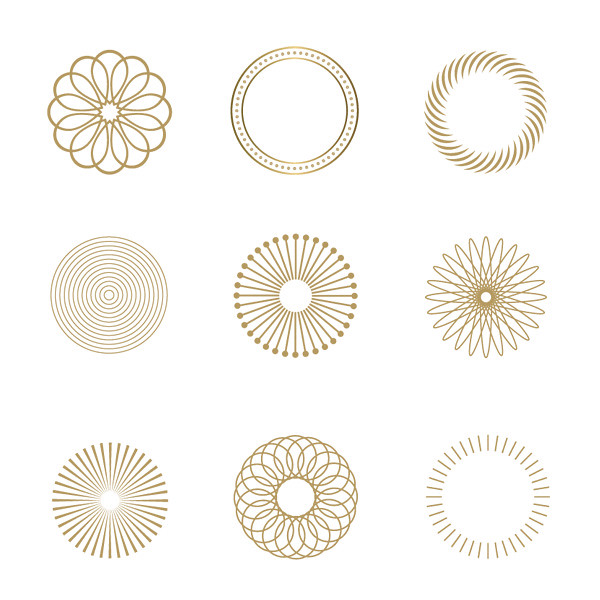This is a graphic featuring nine unique circular designs arranged in a three-by-three grid on a white background. Each circular design is rendered in a brownish-orange or goldish-brown color. The designs vary, including intricate patterns and simplistic forms:

1. The top left design resembles a flower with petal-like spirals.
2. The top middle design features a single band encircling the edge of the circle.
3. The top right design is a banded border that looks somewhat like hair.
4. The middle left design is a spiral pattern.
5. The center design in the middle row has small pins radiating towards the center.
6. The middle right design is another flower, but with pointier leaves.
7. The bottom left design mirrors the pin-like design, but without the tops of the pins.
8. The bottom middle design resembles a donut with squiggly lines around it.
9. The bottom right design consists of straight lines forming a band around the outside of the circle.

Each design is distinct yet cohesive, featuring repetitive motifs and patterns that create a sense of unity within the grid layout.